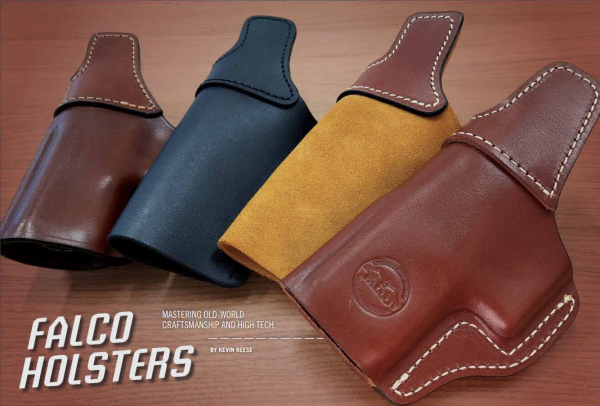The image displays four diverse gun holsters arranged on a wooden table. Each holster features varying colors: the first is brown, the second is navy blue, the third a mustard yellow with a brown strap, and the fourth is a lighter shade of brown. On the lower left side of the image, the brand name "FALCO HOLSTERS" is prominently displayed in italicized, white, all-capital letters. Below a dotted line, there is additional text stating, "Mastering Old World Craftsmanship and High Tech by Kevin Reese," also in white capital letters.